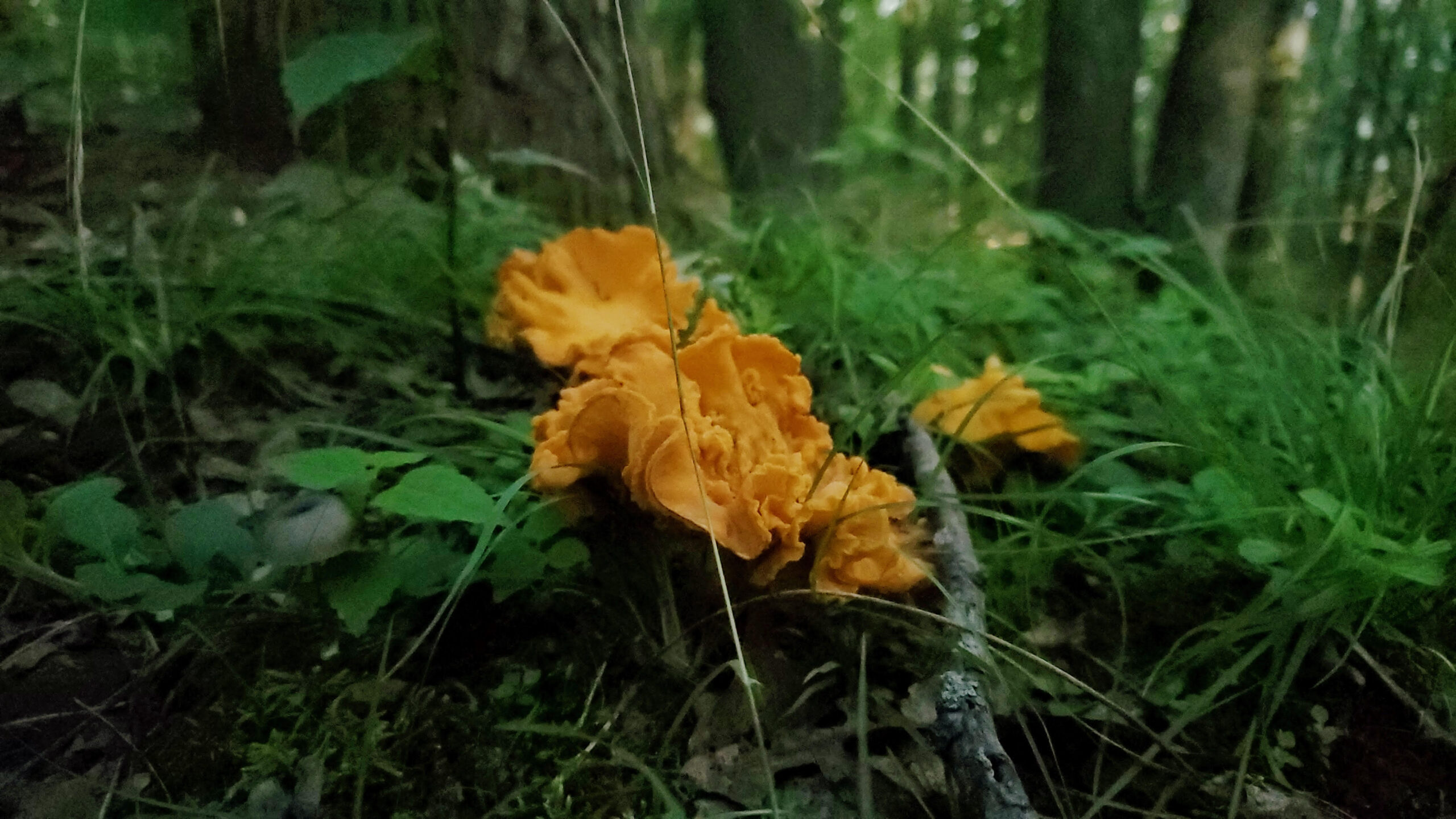The photograph is a detailed, color landscape image capturing a wild chanterelle mushroom as its central subject. This creamy yellowish-orange mushroom, with its ruffled, fan-shaped, and fluffy, flower-like edges, grows prominently from the forest floor, surrounded by lush greenery. Green leaves flank the mushroom on either side, while the foreground is scattered with brown, dried leaves and a twig. Emerging from a wooded area, the image also includes another smaller mushroom to the right of the main cluster. The background reveals a dense forest with visible tree trunks, patches of grass, and a light clearing between the trees, indicating daylight. The overall scene, depicting a natural forest habitat, is captured in a photographic representational realism style.